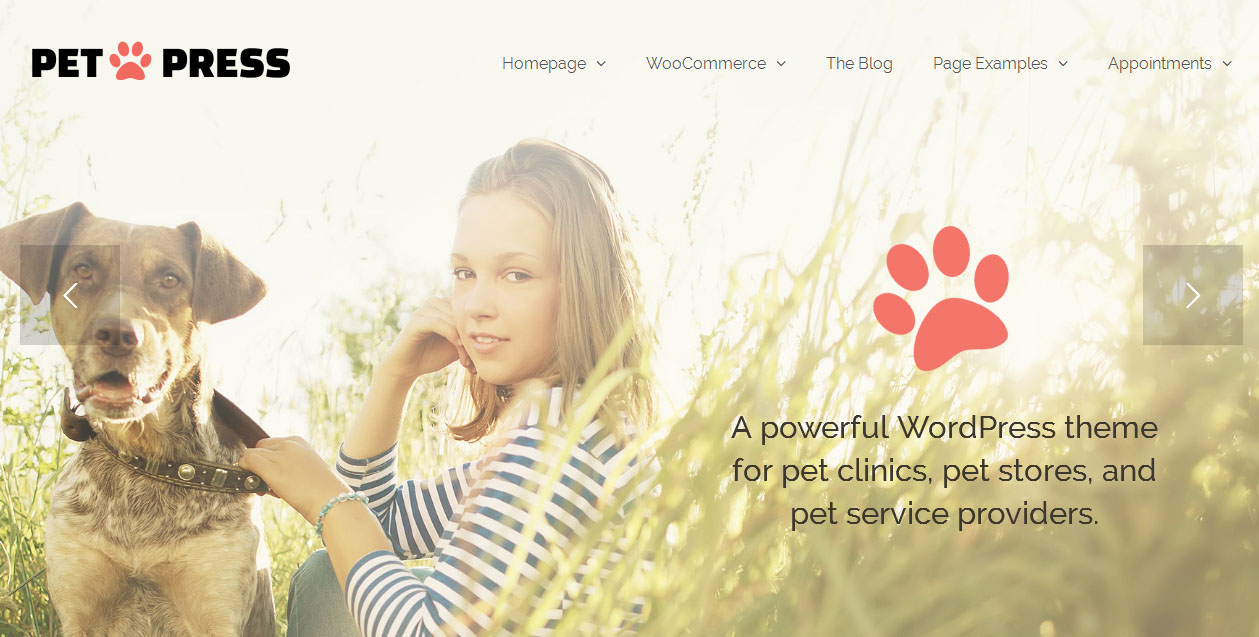In the foreground of a vibrant image set against a yellowish background, a young girl stands holding a brown dog by its collar. They are surrounded by lush grass, creating a serene outdoor setting. In the top left corner, the word "PET" is prominently displayed in black, accompanied by a reddish dog paw print. Below it, the label "PRESS" also appears in black, followed by a series of navigation prompts: "HOME PAGE," "WooCommerce," "BLOG PAGE EXAMPLES," and "APPOINTMENTS," each marked with arrows pointing downwards. Overlaid on the image of the dog are two semi-transparent gray squares; the one on the left contains a left-pointing arrow, while the one on the right has a right-pointing arrow. Adjacent to these squares is a larger depiction of the dog paw print. At the bottom of the image, a bold caption reads, "A powerful WordPress theme for pet clinics, pet stores, and pet service providers," suggesting a versatile and professional theme designed for animal-related businesses.